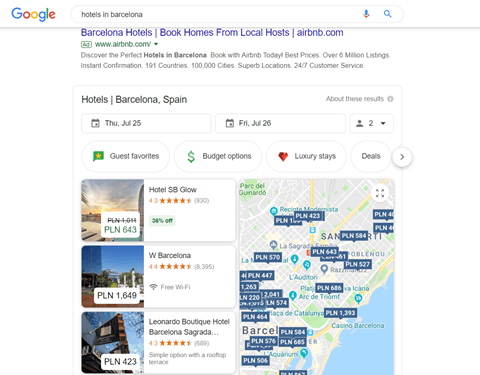This image is a meticulously cropped screenshot from a web page viewed in Google Chrome, excluding any browser or computer interface elements. In the top left-hand corner of the page is the prominent Google logo, adjacent to the search bar where the query "Hotels in Barcelona" has been input. To the right of the search bar are two icons: a microphone and a magnifying glass, the latter representing the search function.

The primary content of the screenshot is focused on the search results for hotels in Barcelona, dated from Thursday, July 25th to Friday, July 26th. At the top of the search results is a sponsored advertisement for Airbnb. Below the ad, Google's search results display a comprehensive list of available hotels on the left-hand side, each entry providing key information such as rates and amenities. Adjacent to this list, on the right-hand side of the image, is an interactive map highlighting the locations of the listed hotels, with markers indicating their exact positions and the corresponding price per night.